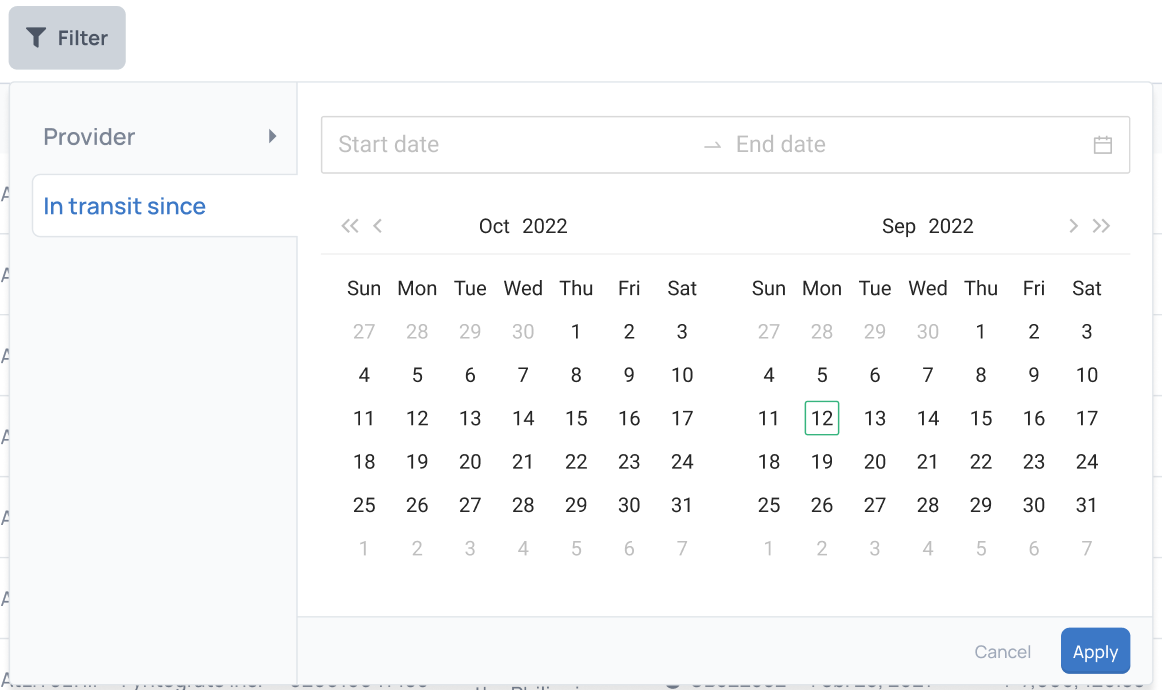In the image, a software interface is displayed prominently. In the upper left corner, there is a button with a filter icon that resembles a funnel. Adjacent to the icon is the word "Filter" against a gray background.

Below this, on the left-hand side, there is a drop-down labeled "Provider" with a small triangle indicating a menu. Further down is a section dedicated to setting date ranges, consisting of two calendar inputs. The top of this section has labels for "Start Date" and "End Date."

To the left of these labels, there are respective calendar icons. The "Start Date" is set to October 2022, and the "End Date" is set to September 2022. Within the calendar, the 12th day of the month is highlighted with a green border around the number '12' in black.

In the lower right corner of the interface are two buttons: a gray "Cancel" button and a blue "Apply" button with white text. These buttons facilitate user actions. Additionally, arrow icons beside the calendars suggest navigation options for selecting different months.